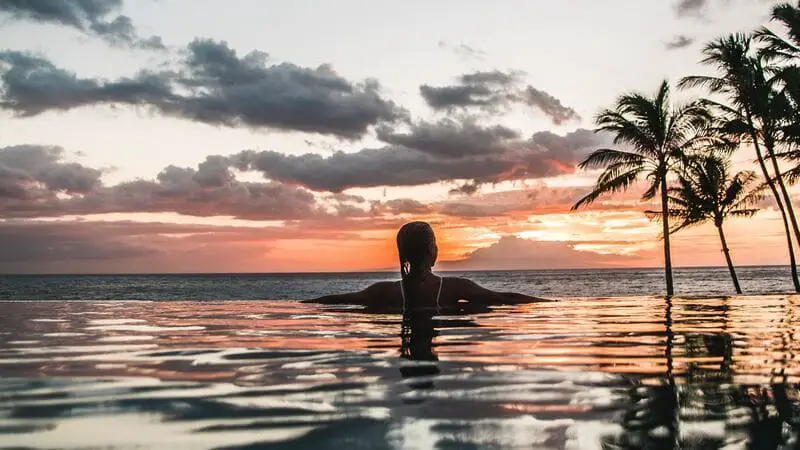This captivating image features a model, partially submerged in an infinity pool, with her back to the camera. Her wet hair cascades down her back as she leans her arms on the faint rim of the pool, gazing towards a breathtaking sunset. The sky is a gradient of gray at the top, transitioning into mesmerizing hues of orange, gold, and pink near the horizon, where a large, puffy cloud partially obscures the sun. These vivid colors are beautifully reflected in the calm, rippling water of the pool, which also mirrors the silhouettes of palm trees to the right of the frame. Beyond the infinity pool's edge, an expansive ocean stretches out, blending seamlessly with the sky, enhancing the serene ambiance of this outdoor scene.